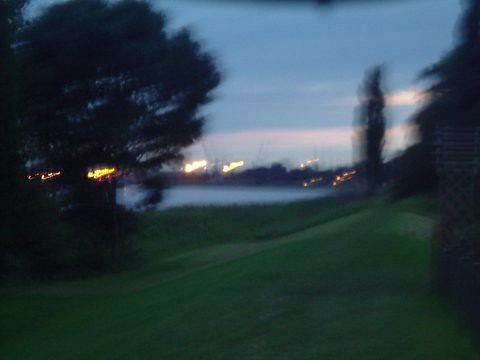Captured in this slightly blurry image is a serene landscape transitioning from day to night. The sky exhibits a beautiful gradient with hues of blue, mingling with touches of purple and pink, signaling the impending dusk. In the foreground, a lush field of green grass gently slopes into a modest hill adorned with verdant trees. A tranquil river meanders through the scene, its calm surface reflecting surrounding lights. Beyond the river, a bridge can be partially discerned, adorned with numerous lights that twinkle like stars. Through the foliage of the largest tree in the frame, clusters of yellow lights can be seen, surrounded by a soft red glow, adding warmth to the setting. Rows of lights across the river illuminate the serene scene, enhancing its peaceful charm.